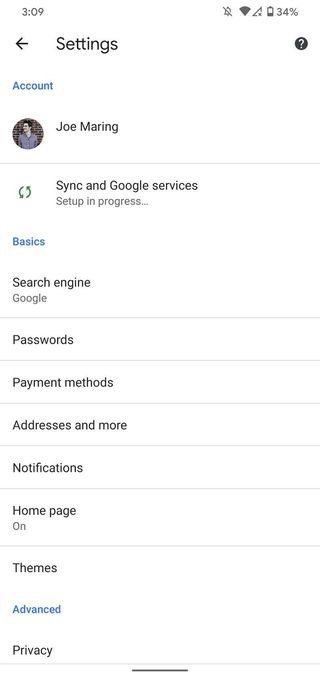The image shows a smartphone screen displaying the Google account settings interface for a user named Joe Marine. 

**Top Section:**
- **Top Left:** The time is 3:09.
- **Top Right:** 
  - A bell icon.
  - Full Wi-Fi signal strength.
  - Cellular signal indicator.
  - Battery at 34%.

**Main Screen:**
- **Left Arrow:** Indicates a back navigation option.
- **Settings Icon:** Represents access to settings.
- **Question Mark in Circle:** Likely for help or support.
- **Avatar:** Displays a user's face, labeled "Joe Marine."
- **Refresh Symbol:** For syncing or refreshing.
- **Sync and Google Services:** Setup is in progress.

**Sections & Options:**
1. **Basics**
2. **Search Engine:**
   - Set to Google.
3. **Passwords:** Option presumably for managing saved passwords.
4. **Payment Methods:** For managing saved payment details.
5. **Addresses and More:** Likely for address management.
6. **Notifications:** For managing notification settings.
7. **Homepage On:** Indicates that the homepage setting is active.
8. **Themes:** Option for customizing the theme.
9. **Advanced:**
   - Under a small blue text label.
10. **Privacy:** Another section further listed.

The overall screen is dedicated to fine-tuning various settings related to the user's Google account, with detailed options for security, personalization, and service preferences.